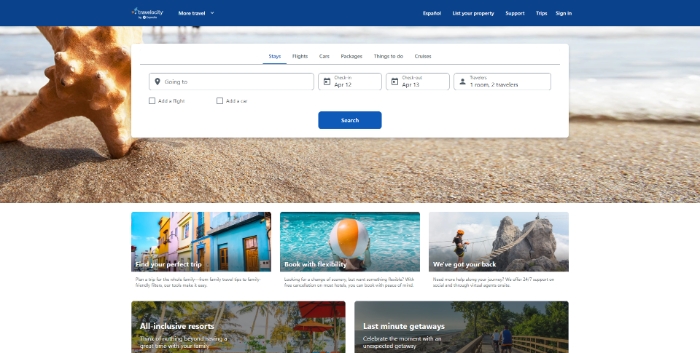The image is a screenshot showcasing the home page of a travel booking website, specifically Travelocity. At the top, a blue header prominently displays the Travelocity logo on the left, accompanied by their slogan. The header also includes various navigation options: "More Travel," "Español," "List Your Property," "Support," "Trips," and "Sign-In." 

Directly below the header is a comprehensive search bar with tabs for different travel options: "Stays," "Flights," "Cars," "Packages," "Things to Do," and "Cruises." The search bar includes fields for destination input ("Go-To"), check-in and check-out dates, and number of travelers, along with additional options to add a flight or a car. A prominent blue search button is centrally positioned.

The background behind the search bar is a serene beach scene featuring sand and a large starfish on the left side, with the ocean visible in the background, enhancing the travel theme.

Beneath the search bar and background image, several featured sections promote various travel services, including:

- "Find Your Perfect Trip"
- "Book with Flexibility"
- "We've Got Your Back," which displays an image of two people hiking on rocks and includes a note about 24/7 support.

Additional sections include:

- "All-Inclusive Resorts," featuring an image of a resort with palm trees and information about all-inclusive deals.
- "Last-Minute Getaways," highlighted by an image of a person walking on a wooden bridge and details about spontaneous travel offers.

The overall design is clean and user-friendly, focusing on the search functionality at the top. Vibrant and inviting images emphasize the travel destinations, predominantly featuring shades of blue consistent with the theme.